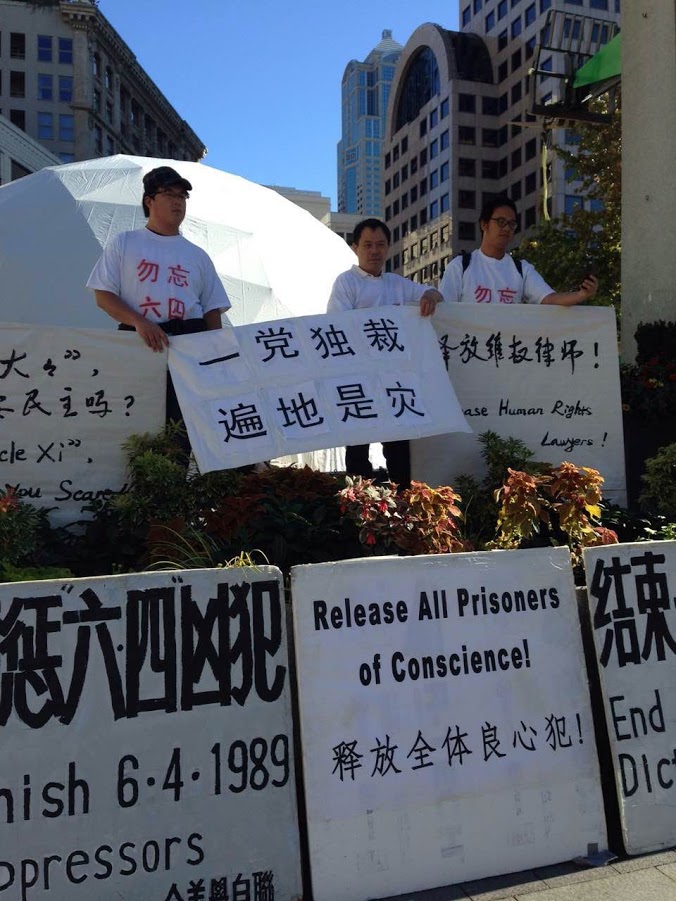In this image, three Asian men stand prominently on a small elevation, possibly a wall, against the backdrop of a partial globe structure. All three are dressed in white shirts; the middle individual wears a polo shirt while the others sport regular white tees. The man on the left accessorizes with a black hat and glasses, the man in the middle is without headgear, and the man on the right wears glasses.

They are holding protest signs adorned with black symbols and East Asian script, likely Chinese. The two men on the left and in the middle are holding a rectangular banner with eight symbols, arranged four on top and four on the bottom. Additional signs are placed on the sidewalk below, propped against a wall, featuring English text and the script. One sign implores, "Release all prisoners of conscience," highlighting a plea for human rights. Another sign references the date "6-4-1989," indicative of a significant historical event, and yet another calls to "End Dictatorship," while urging the support of "human rights lawyers." The setting appears to be an urban area, possibly in China or Hong Kong, and the scene suggests an organized protest advocating for political freedom and human rights.